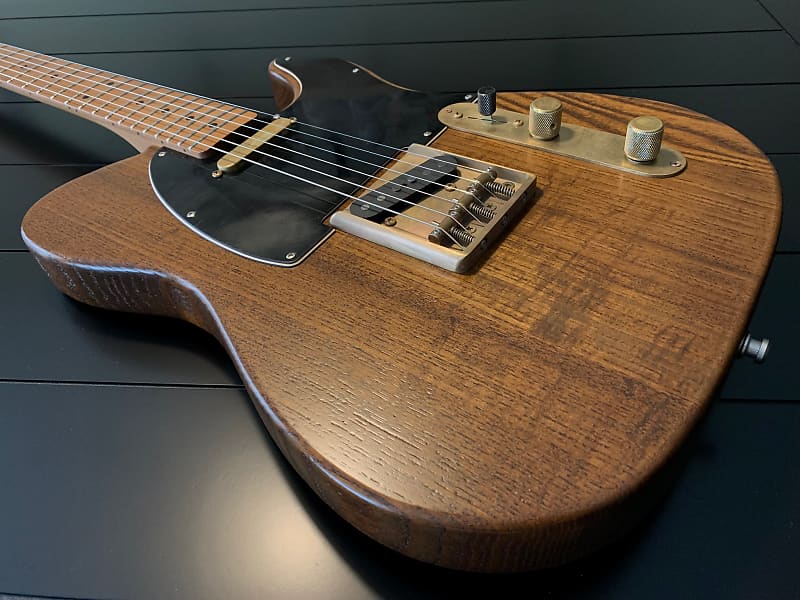This exceptionally high-resolution professional photograph captures a modern electric guitar displayed against a glossy black background. The guitar itself, crafted from a solid, thick slab of what appears to be oak or walnut wood, showcases a beautifully polished and stained finish that highlights its natural wood grain. It features six silver strings and a variety of controls, including volume knobs made of either chrome or brass. The guitar's design emphasizes simplicity and craftsmanship, forgoing flashy colors in favor of a classic, natural aesthetic. A black guard, possibly metal or plastic and secured with screws, lies under the fretboard, adding a touch of contrast. This intricately detailed close-up, with its sharp focus and rich textures, portrays an instrument that is clearly cherished and meticulously maintained, likely considered the owner's pride and joy.